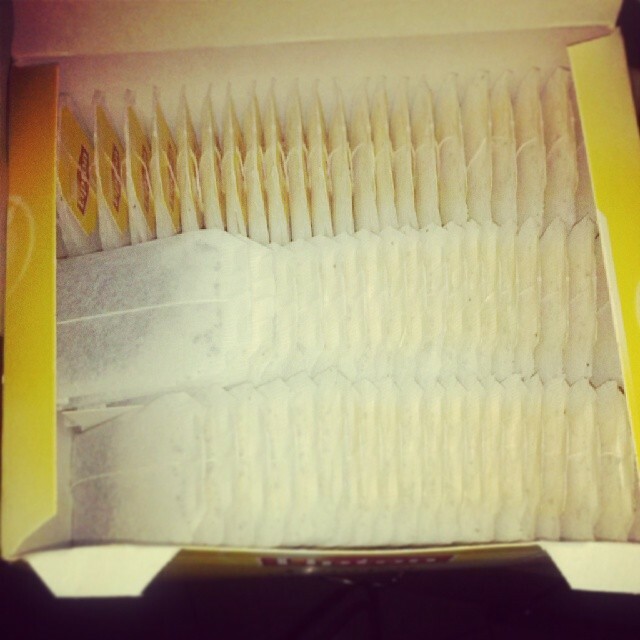The image depicts an open box of Lipton iced tea bags, characterized by its yellow exterior and white interior. The box contains three rows of mini tea bags, each row holding approximately 15-20 white tea bags adorned with the yellow and red Lipton logo. The tea bags are neatly arranged, with some rows lying flat and the last row standing upright, indicating minimal usage. Strings attached to the tea bags run along the sides, and the semi-transparent bags reveal dark tea within. The box is placed on a dark, possibly purple, background, accentuating the organized presentation of the tea bags within.